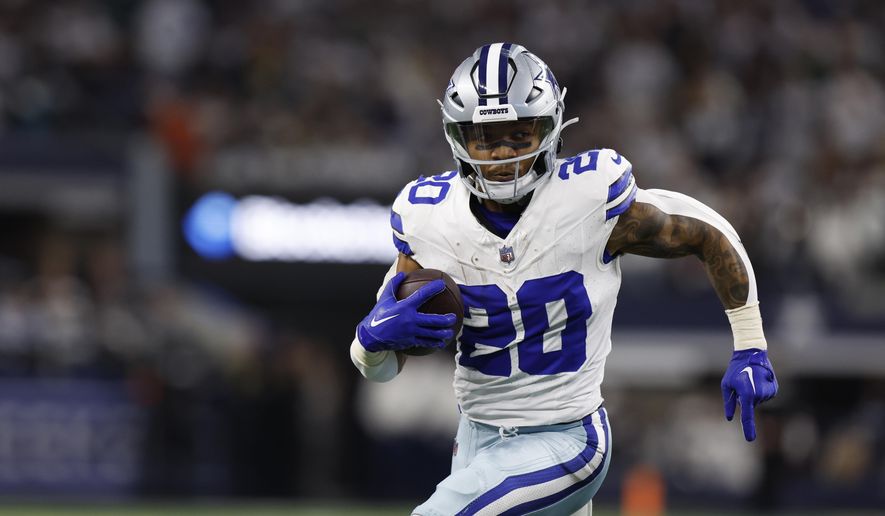In the foreground of the image, a Dallas Cowboys football player is captured mid-motion, running slightly to the right and facing forward. He is sporting a white jersey adorned with royal blue lettering and the number 20. His helmet is silver with a navy and white stripe, and it also features the word "Cowboys" on a small strip in the front. His face bears a black strip over his nose and under his eyes.

The player's attire includes blue and white gloves with the Nike logo, light blue pants accented with a blue and white stripe, and white strips on his arms and wrists. He is holding an American football in his right hand while his left hand swings backward, and his left leg moves forward as he runs.

The background is a blurred view of what appears to be a stadium filled with people. Although the details are indistinct, there's a suggestion of stadium seating, neon lights, and possibly a goalpost, all contributing to the sense of a lively game setting.